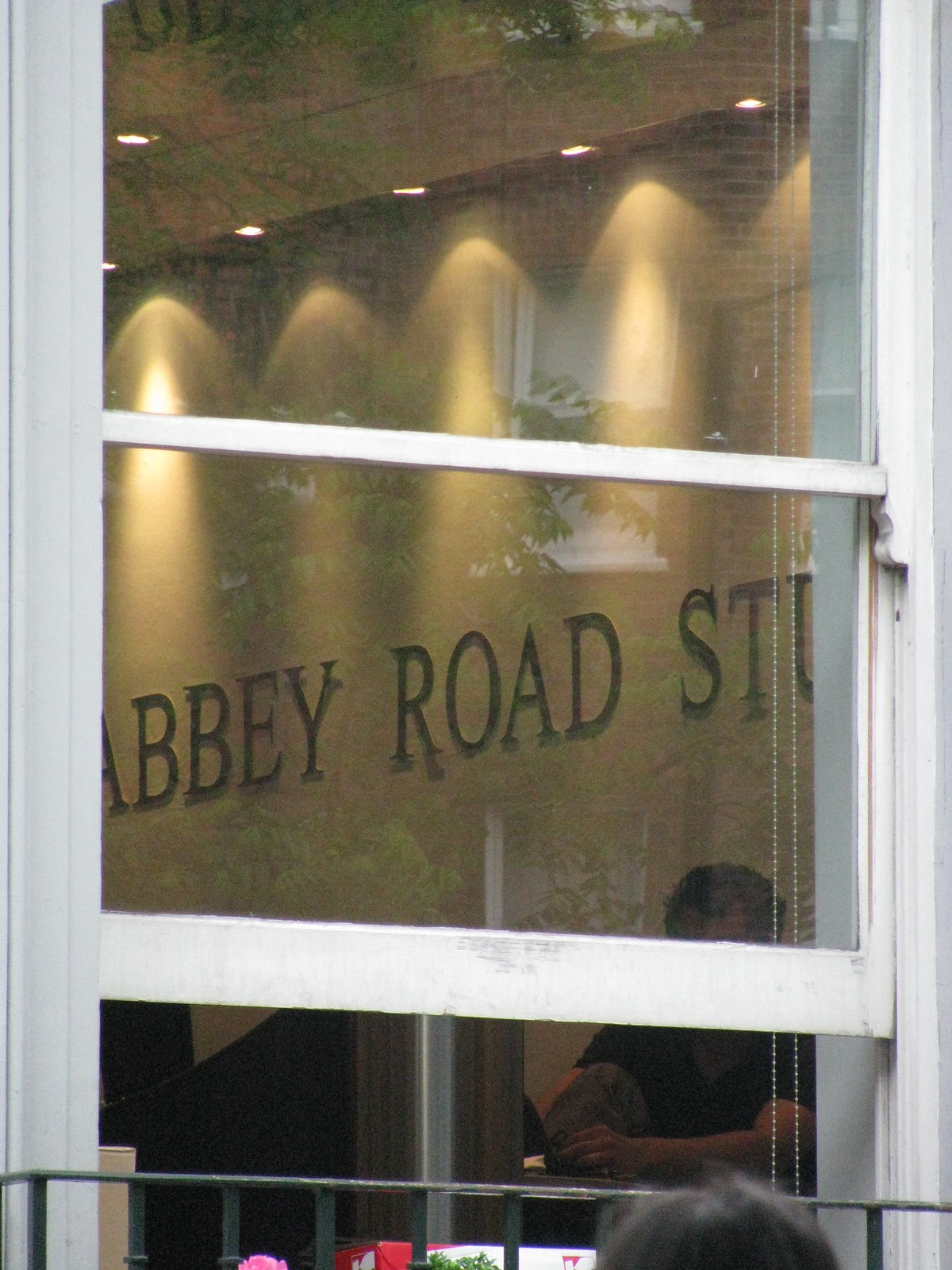The image is a color photograph in portrait orientation capturing an exterior view into the interior of a building, likely a studio lobby, through a slightly open, white wood-framed window. Reflections on the glass reveal trees and an additional window inside the building. Prominently displayed on the pale gold interior wall is a sign with spotlights illuminating the text "Abbey Road STU," likely referring to "Abbey Road Studio." Within the room, several individuals are visible, either seated or potentially standing, while a black-haired person is in the bottom right foreground looking through a black wrought iron gate. The scene includes touches of colors such as pink flowers, red tones, and various shades of white, black, and gray, suggesting it was taken during the daytime. The style is a realistic photographic composition.